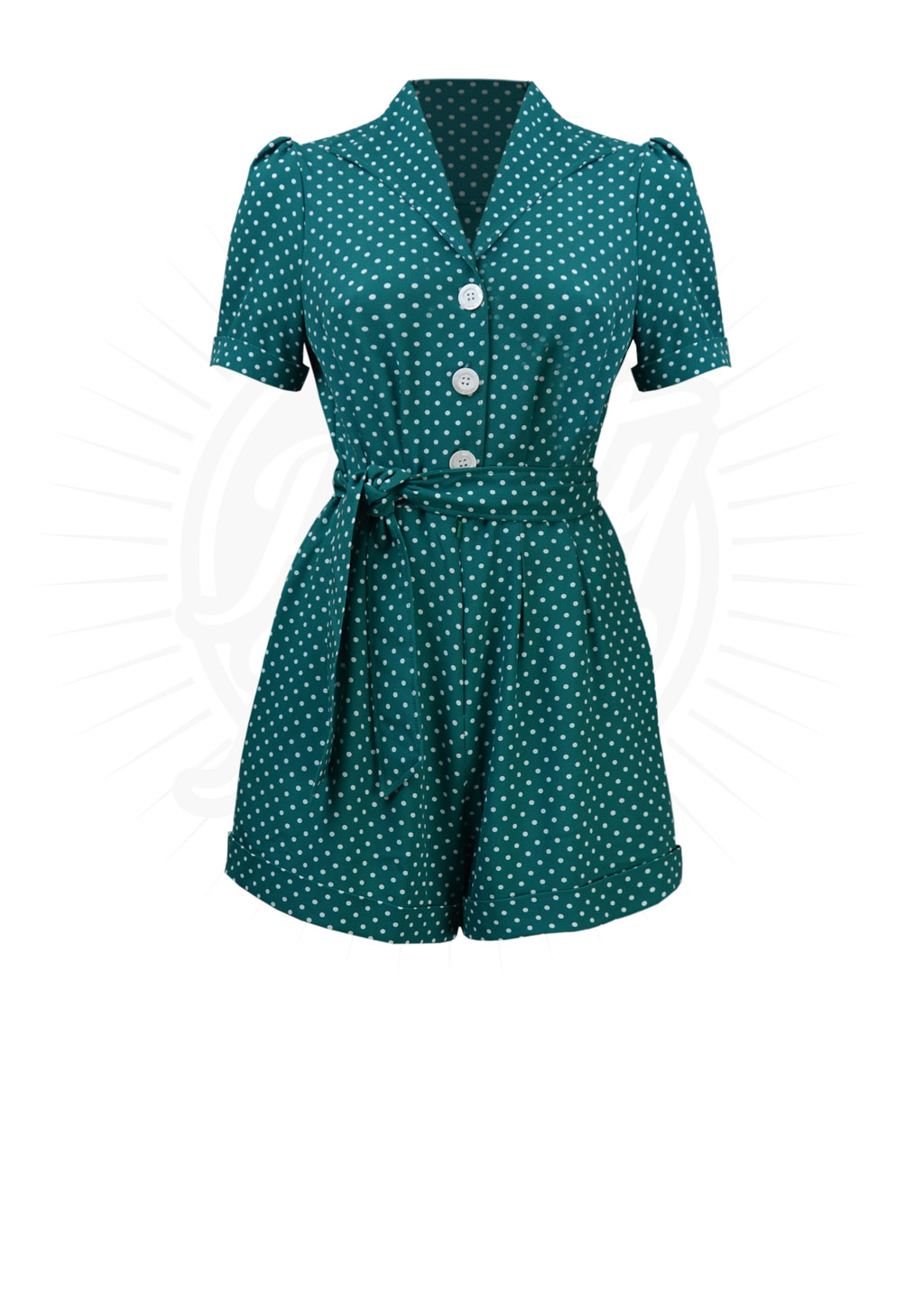This product image features a vintage-style teal jumpsuit adorned with white polka dots. The outfit boasts a fitted bodice accentuated with darts and a V-shaped neckline, complemented by a lapel collar. Three prominent white buttons secure the front, while a waist tie adds a touch of sophistication. The short, slightly gathered sleeves end in neat cuffs, matching the pleated shorts, which also feature cuffs and fall just above the knee. This one-piece romper design evokes a sense of timeless fashion. The pristine white background highlights the garment, adding emphasis to its details, and in the backdrop, a light gray watermark with sunrays subtly appears, possibly indicating the brand or a stock photo insignia.